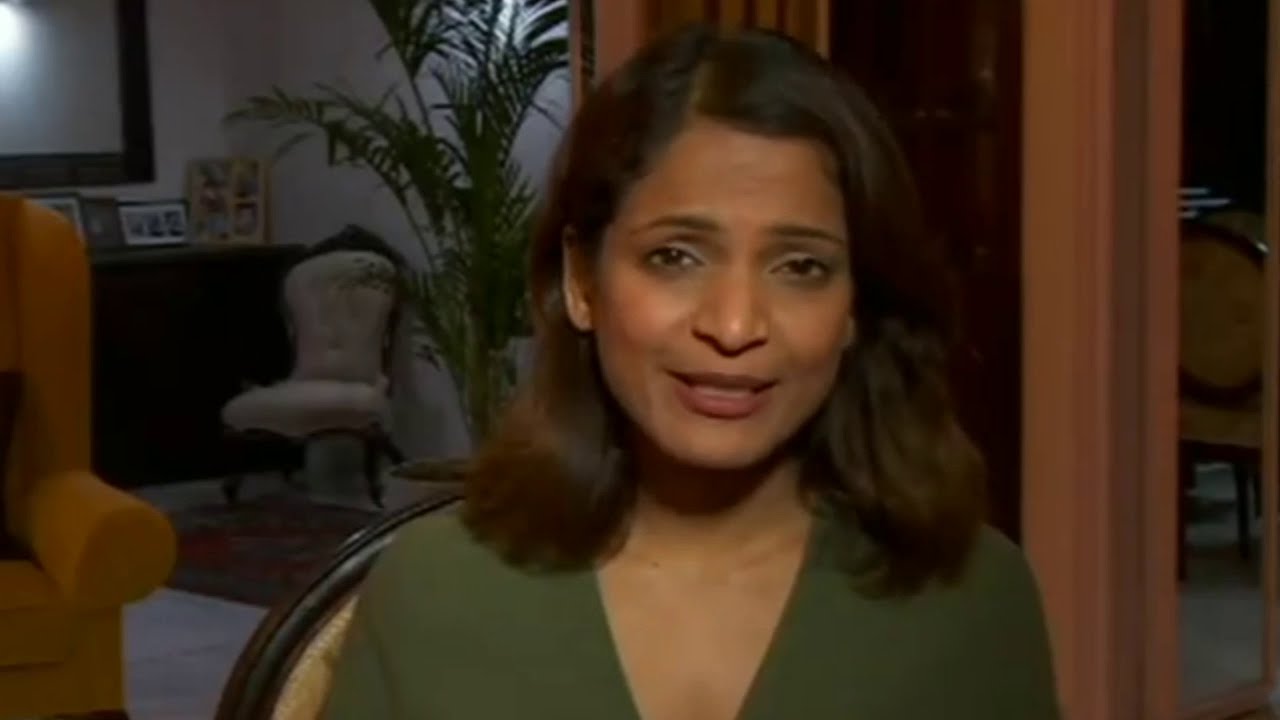This photograph captures a woman, who appears to be between 35 to 40 years old, with medium-dark skin and shoulder-length dark brown hair adorned with reddish highlights. She is gazing forward at the camera, her mouth slightly open as if speaking, revealing her bottom teeth. She has red lips and a squint in her eyes, creating an expression that exudes both focus and warmth. She is dressed in an olive-colored top with a low-cut V-neck. 

The setting appears to be a cozy, elegantly furnished room, potentially a living area in a house. The backdrop features a variety of details: to the woman's right, there is a striking orange armchair, and further to the right in the corner is a large mirror with a wooden frame hanging on a gray-painted wall. Below the mirror sits a dresser or cabinet adorned with framed photographs. To the adjacent side of this cabinet, an antique chair or table sits upon a Persian rug next to a sizable palm plant in a pot. To the woman's left, there are glass doors that add light and dimension to the room. The overall setting, with its mix of modern and antique elements alongside vibrant plants, provides a rich, detailed context that complements the woman's composed yet engaging presence.